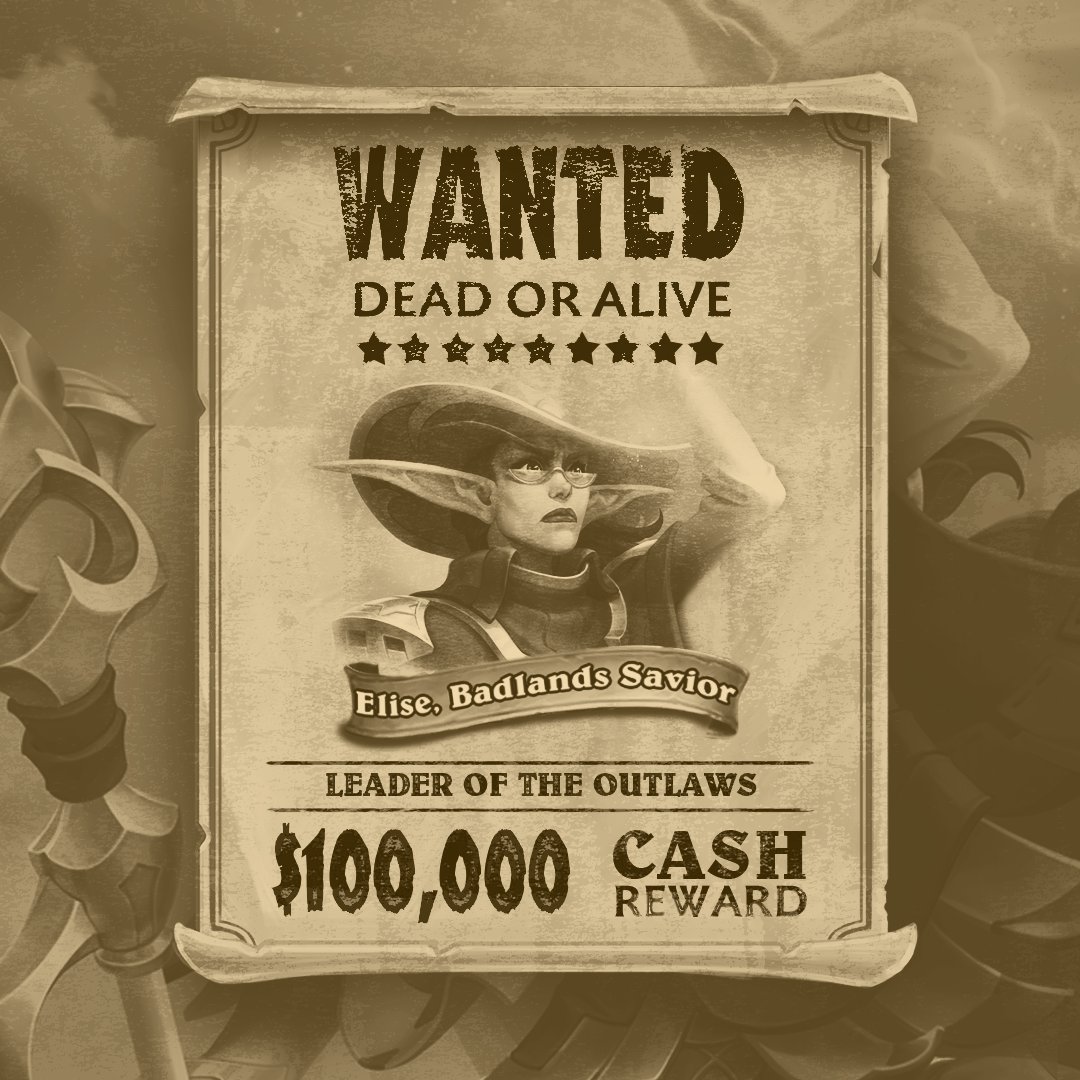The image is a detailed, computer-generated wanted poster set in a fantastical, western-themed environment. Dominated by various shades of brown and black to evoke an antiquated, almost sepia-tone feel, the background features a dark beige or khaki color, enhancing the vintage aesthetic. Prominently displayed in the foreground is the wanted poster, which reads in bold, dark brown letters at the top: "WANTED, DEAD OR ALIVE." Beneath the heading, a portrait of a female elf with extremely long and pointy ears wears a large witch or cowboy hat, complemented by small bifocals perched on her nose. She dons a black cape or suit and stands with her left hand raised, looking towards the right side of the image. The text further describes her as "ELISE, BADLANDS SAVIOR" and "LEADER OF THE OUTLAWS," with a "100,000 CASH REWARD" offered for her capture. The background includes various elements like a metallic staff or scepter on the left-hand side and possibly some armor or clothing on the lower right, adding to the scene's depth and reinforcing the blend of fantasy and western motifs commonly found in digital artwork or video games.